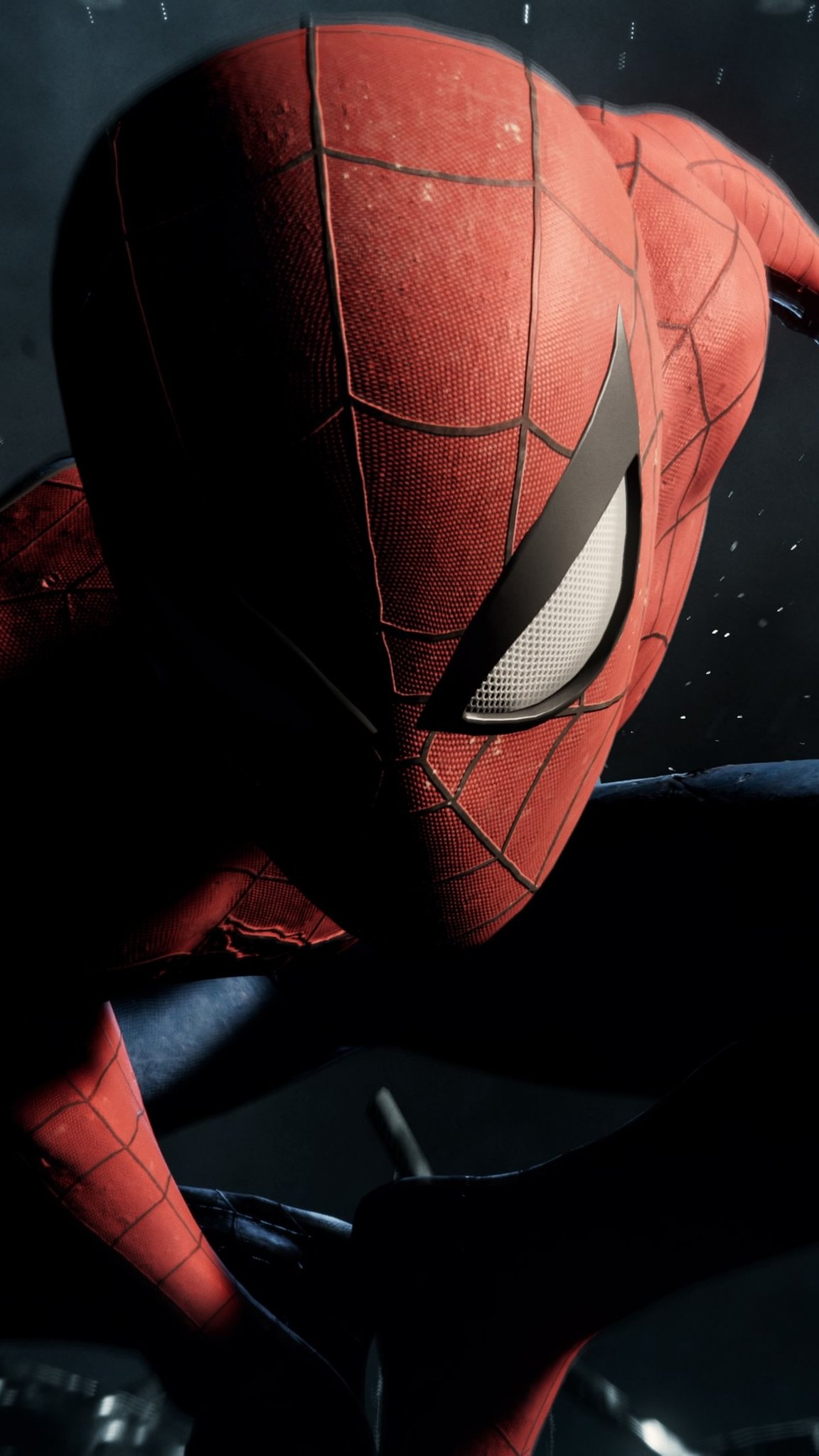Spider-Man, clad in his iconic red suit, stands heroically. His suit is adorned with intricate black markings that resemble spiderwebs, stretching across his face, shoulders, and arms. The eyes of his mask are outlined in a black rubber-like material, with a luminous center that features small perforations, allowing visibility. Below, there is a dark area suggesting he is either landing or perched on a surface made from a plastic-like fabric. The overall effect captures the detailed and dynamic design of Spider-Man's attire in a dramatic setting.